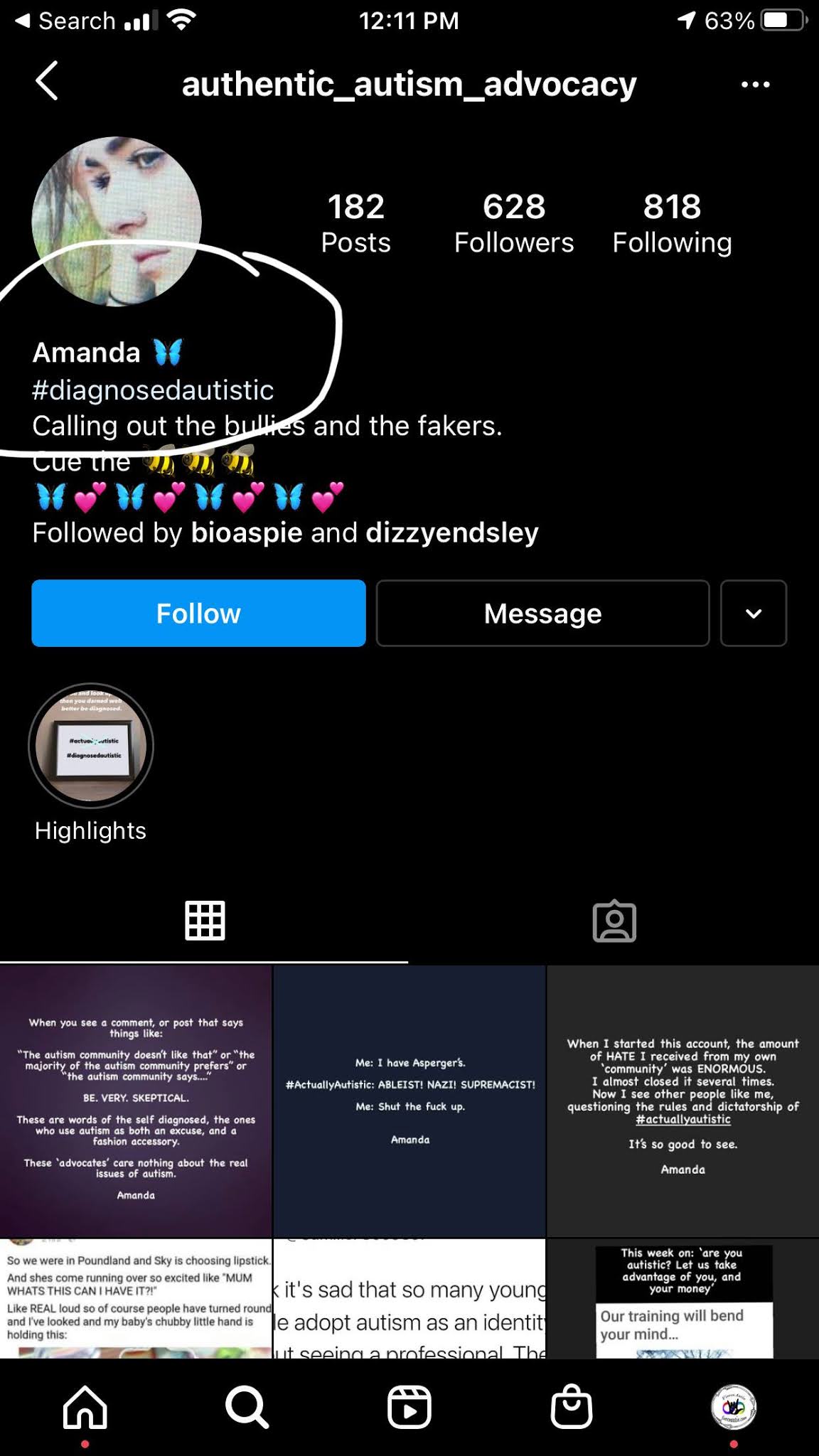The image is a screenshot of a Twitter profile on a smartphone. At the very top, the phone's status bar shows a Wi-Fi icon, the time (12:11), and the battery life at 63%. Below that, it is evident that the app in use is Twitter. The profile has 182 posts, 628 followers, and is following 818 accounts. 

To the left of these statistics is a circular profile picture of a user named Amanda, accompanied by a butterfly emoji. Her bio reads, "Hashtag Diagnosed Autistic" followed by the phrase "Calling out the bullies and the fakers" with three bee emojis in succession, and additional butterfly-heart emoji pairs.

The profile indicates it's followed by several users and presents options to either follow, message, or access additional actions via a dropdown box. Beneath the follow button, there's a "Highlights" section depicted with a circular thumbnail.

The main content area displays a grid of six text-based quotes that Amanda has posted, organized in two rows with three quotes each. One of the quotes advises caution against believing statements like, "Autism community doesn’t like that," urging viewers to be skeptical. Another quote discusses Amanda's experience with Asperger's. 

At the bottom of the screen, there are five navigation icons: Home, Search, Notifications, Shopping, and Profile.